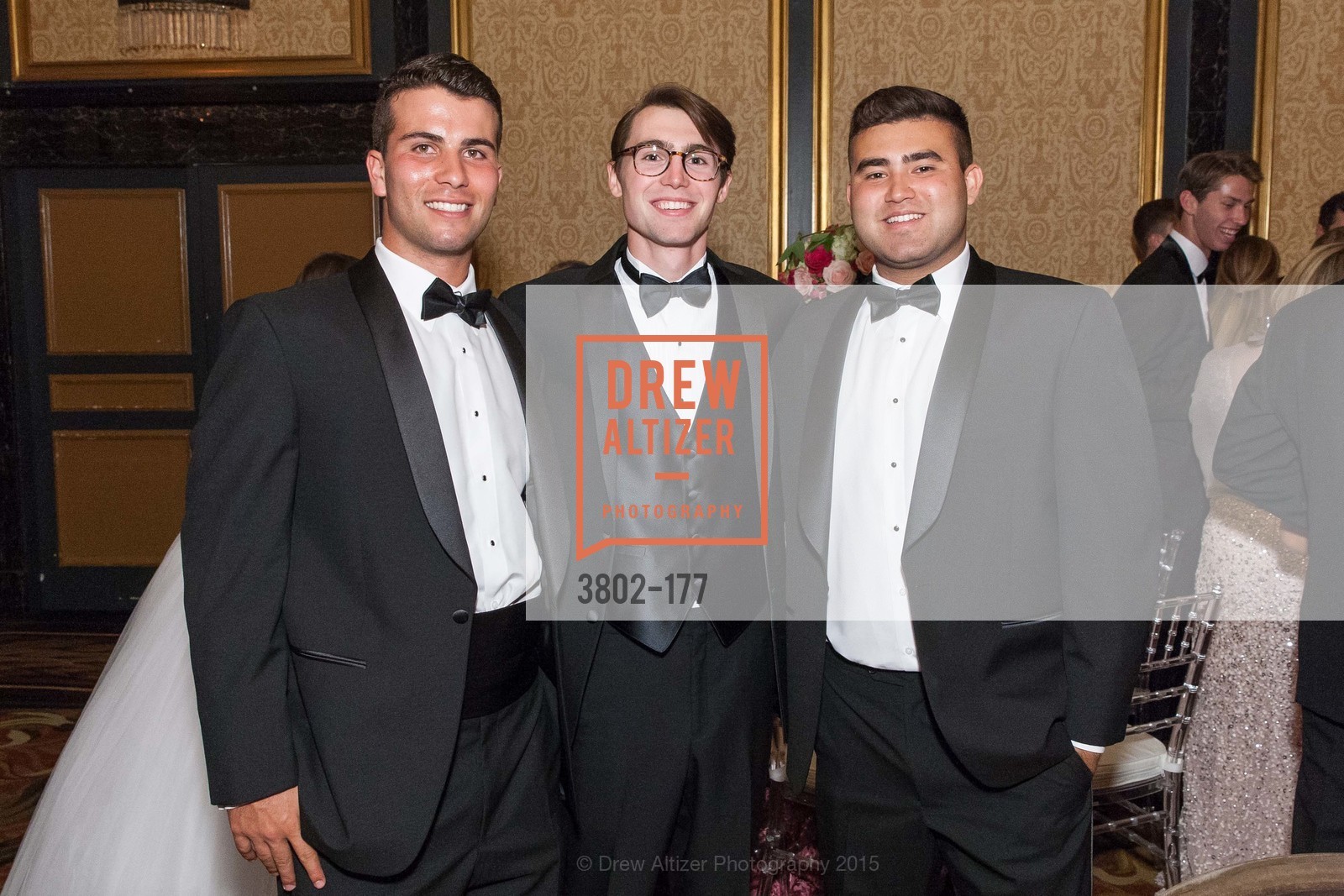In the photograph, three smiling men stand close together, dressed in elegant black tuxedos with white shirts and black ties. The man on the left is a white male with dark hair, not wearing eyeglasses. The man in the middle, also a white male, wears eyeglasses and a tuxedo. The man on the right, who appears to be either Latino or Asian, sports a similar short dark hairstyle and tuxedo. They seem to be in their early to mid-20s. In the background, a group of other young men and women are also dressed formally, with people in tuxedos and dresses, hinting at a fancy banquet or possibly a wedding in a ballroom or convention hall. The venue features a patterned wall with blue stripes. The image is watermarked with "Drew Altizer Photography" and includes a reference number "3802-177," along with a copyright notice for Drew Altizer Photography from the year 2015.